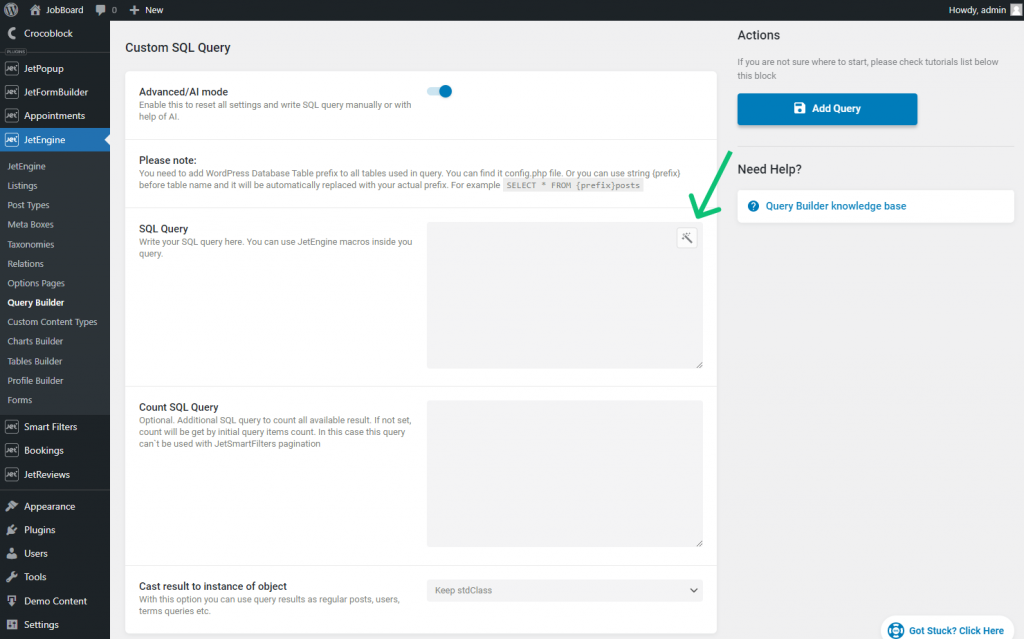The image is a screenshot depicting a web page, prominently featuring a black header at the top with the text "Job Board." Beneath the header, there is a navigation menu labeled "Crocoblock," which lists various tools and features. The menu includes "Jet Popup," "Jet Form Builder," "Appointments," and multiple entries for "Jet Engine" followed by subcategories such as "Listings," "Post Types," "Meta Boxes," "Taxonomies," "Relations," "Options Pages," "Query Builder," "Custom Content Types," "Charts Builder," "Tables Builder," "Profile Builder," "Forms," and continues with "Smart Filters," "Bookings," and "Jet Reviews." Further down the menu, additional options include "Appearance," "Plugins," "Users," "Tool," "Demo Content," and "Settings."

To the right of this menu, the larger, white main section of the page displays various SQL-related functionalities. This section includes headings like "Custom SQL Query," "Advanced AI Mode," "SQL Query," "Count SQL Query," and "Cast Result to Instance of Object." On the far right of this section, there is an "Actions" column featuring a prominent blue button labeled "Add Query."